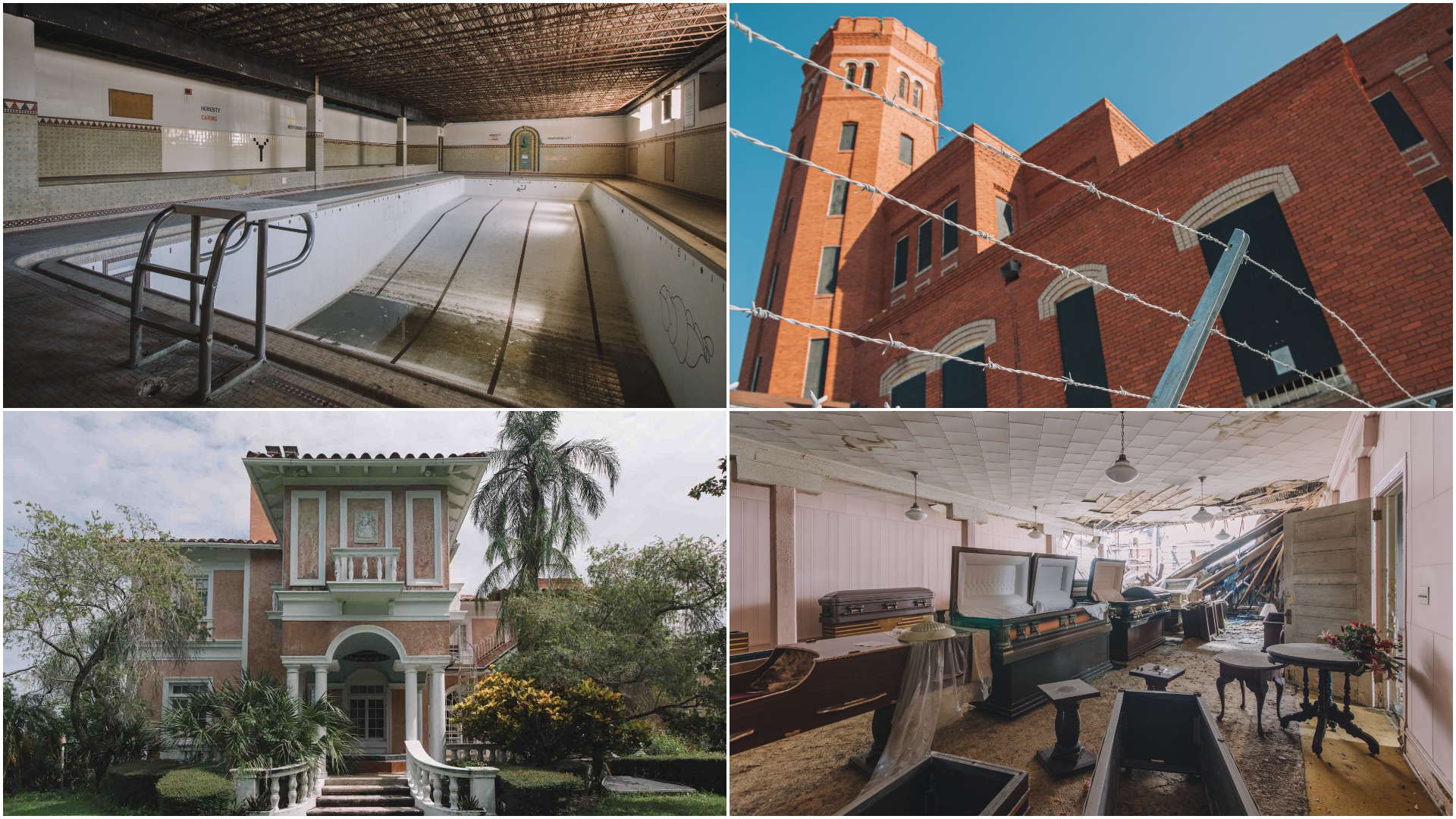This image is a collage of four distinct views showcasing different areas of various buildings. In the top left, we see the interior of a large, drained swimming pool room. The area includes big walls, a brown roof, an entrance door, columns, and stairs leading to what might once have been the diving platform. The top right image displays the exterior of a grand, modern brick building with large black windows, bathed in sunlight against a clear blue sky; barbed wire appears to surround it. The bottom left photo shows a two-story, grand bungalow with a smooth, potentially marble exterior, featuring an entrance with white railings, pillars, and a staircase, with a balcony above and a garden surrounding the premises, all illuminated by daylight. The bottom right image reveals a decrepit room possibly used as a funeral home; it has broken walls and ceiling, battered furniture, coffins in various states of disrepair, ceiling fans, tables adorned with flowers, and an open door, contributing to its worn-out appearance.